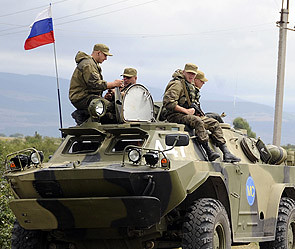The image depicts a Russian military armored vehicle in an outdoor setting, prominently positioned in the foreground. Four soldiers, dressed in military uniforms complete with hats and army boots, are sitting atop the camouflaged vehicle. Each soldier appears relaxed, holding guns as they ride the armoured car. Notably, the vehicle features large black tires and has a blue circle with the letters "MC" painted on the side. A Russian flag, displaying the colors white, blue, and red, is attached to this military vehicle. In the background, a cloudy, overcast sky stretches above a series of hills and mountains, with an electricity pole and wires faintly visible to the right. The terrain around the vehicle is dotted with green grass, contributing to the overall atmosphere of an operational military scene.